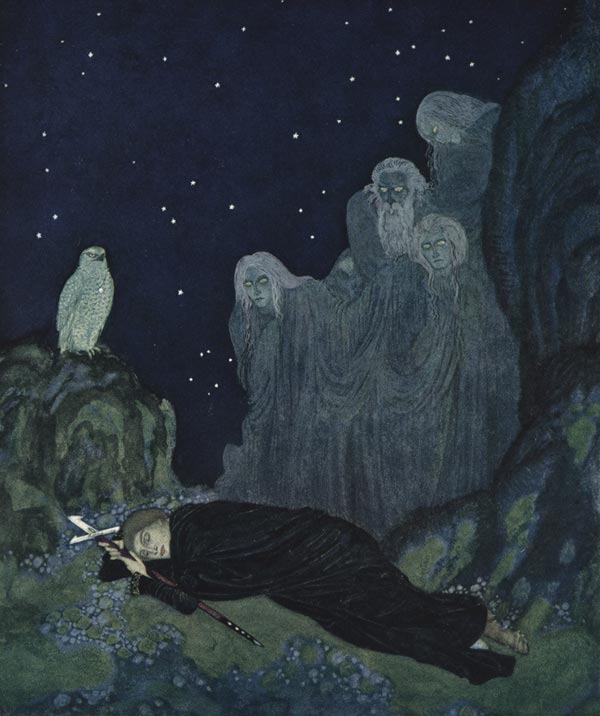In this dark, monochromatic painting, a monk-like figure is depicted sleeping on their right side, their head resting on an arm, and holding a staff with a cross at the top. They're positioned at the bottom of the image, nestled amidst greenish-gray rocks and boulders that form a rugged landscape. The scene is set under a black sky dotted with white, giving a nightmarish ambiance. On the left, atop a rocky structure, a bird of prey, possibly an eagle or owl, gazes toward the background. To the right of the monk, emerging from the stone formations, are four ghostly, gray figures with haunting white eyes and diverse hairstyles, draped in a single, eerie fabric. These figures, reminiscent of the dead, seem to watch the sleeping monk intently, adding to the painting's eerie and mystic feel.